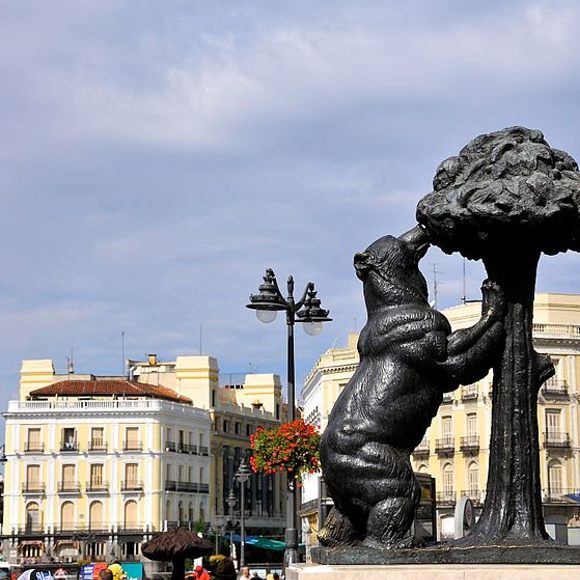This vibrant cityscape photograph, likely set in a European city boasting old-style architecture, features a striking statue of a black bear. The bear, crafted from iron, stands on its hind legs, apparently sniffing or licking the leaves of a tree situated on its right side. This statue occupies the lower left to middle portion of the image. The urban backdrop shows predominantly white, multi-story residential buildings that hint at a French architectural influence. Adding a touch of charm, a light post with an array of flowers adorns the center of the scene. The sky is a very light blue with scattered clouds, indicating a bright day. The colors throughout the photo range from black and white to an assortment of vibrant hues, including red, green, blue-green, yellow, orange, beige, and a very light yellow, enriching the overall visual narrative.